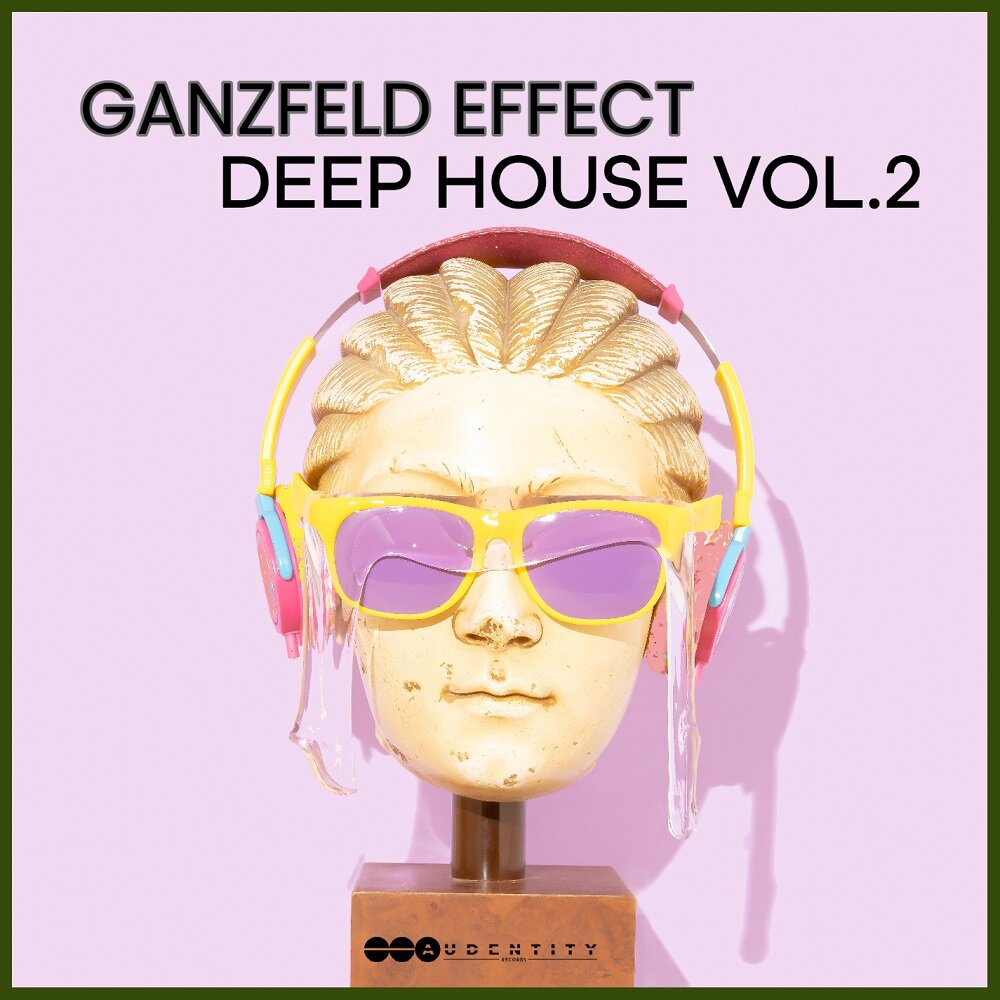This image is a poster-like painting, possibly an album cover, with the main focus being on a beige-colored mannequin head adorned with vibrant accessories. It features a square layout, framed by a thick dark green or black border. The background of the square is predominantly lavender or light pink.

At the very top of the image, in large, bold black letters with a dark grey outline, the text reads "Gansfeld Effect, spelled G-A-N-Z-F-E-L-D Effect." Directly underneath, in slightly less bold black letters, it says "Deep House, Volume 2."

The mannequin head, positioned in the center, has tight, cornrow-style braids and is accessorized with yellow-framed sunglasses featuring lavender or opaque purple lenses. It also wears colorful headphones, predominantly yellow, pink, and light blue in color. The head is mounted on a little wooden or marble stand.

At the base of the stand is a logo or text that reads "A-U-D-E-N-T-I-T-Y Records" or "Identity." The overall composition of the image combines a retro aesthetic with modern elements, creating a visually striking representation.